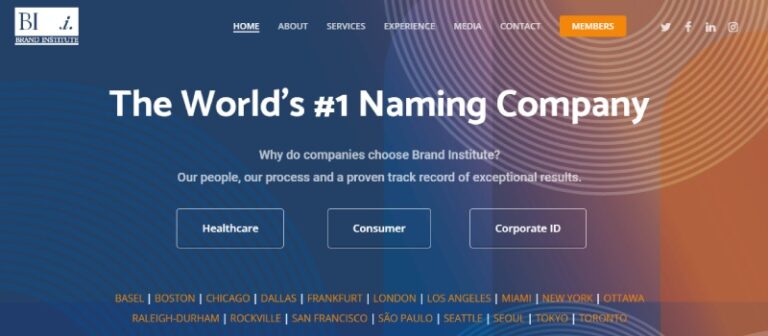The image depicts a website with a sleek, blue-themed design, belonging to an unidentified institute abbreviated as "BI." 

In the upper left corner, there is a distinctive white rectangle featuring blue text with the "BI" acronym prominently displayed. Across from this logo, the website hosts a series of drop-down menus including: Home, About, Services, Experience, Media, and Contact. 

Adjacent to these menus, there is an orangish-yellow button labeled "Members," which allows users to sign in for premium content. Towards the right edge of the page, there are social media icons for Twitter, Facebook, and Instagram, providing quick links to the institute's social media profiles.
 
Centrally displayed across the website is a bold slogan proclaiming, "The World's Number One Naming Company." This tagline suggests the institute specializes in the field of naming, asserting itself as the leading entity in the industry.